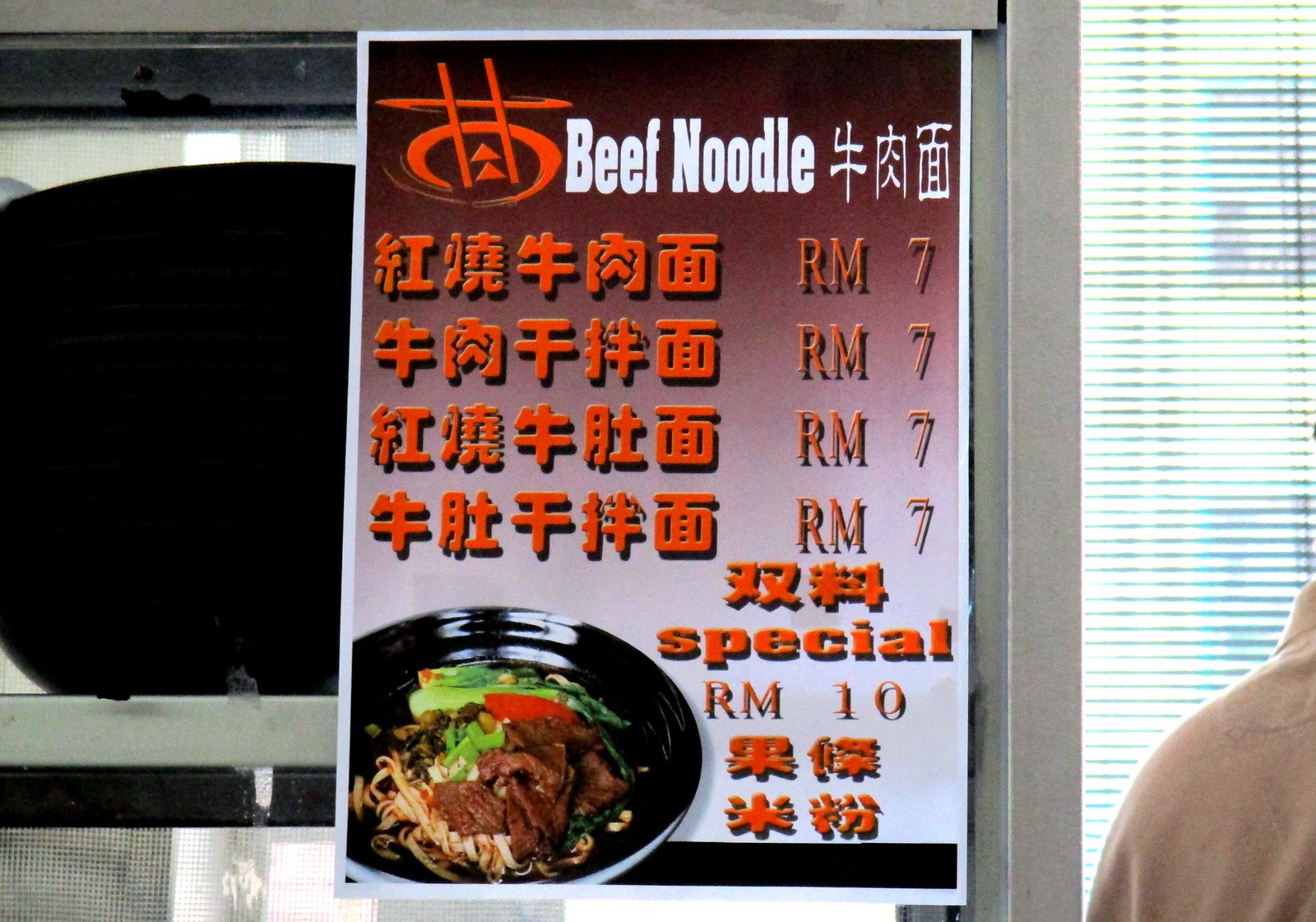The image depicts a restaurant menu poster displayed on a window, written predominantly in Asian characters. The menu has a gradient background that transitions from a darker red-maroon at the top to pink and finally white at the bottom. Prominently, at the top, "Beef Noodle" is written in white English letters alongside similar Asian characters. Below this title, four lines of red Asian text enumerate various dishes and prices, with RM7 frequently appearing. Towards the bottom, the menu highlights a "Special" priced at RM10 with accompanying characters. The poster also features a large black bowl filled with sliced steak, noodles, and vegetables. Partially visible to the right of the image is someone's shoulder in a white shirt, standing in front of a window or door with an open shade, letting in some light. Likely, behind the poster is the restaurant's sign facing outside to inform potential customers.